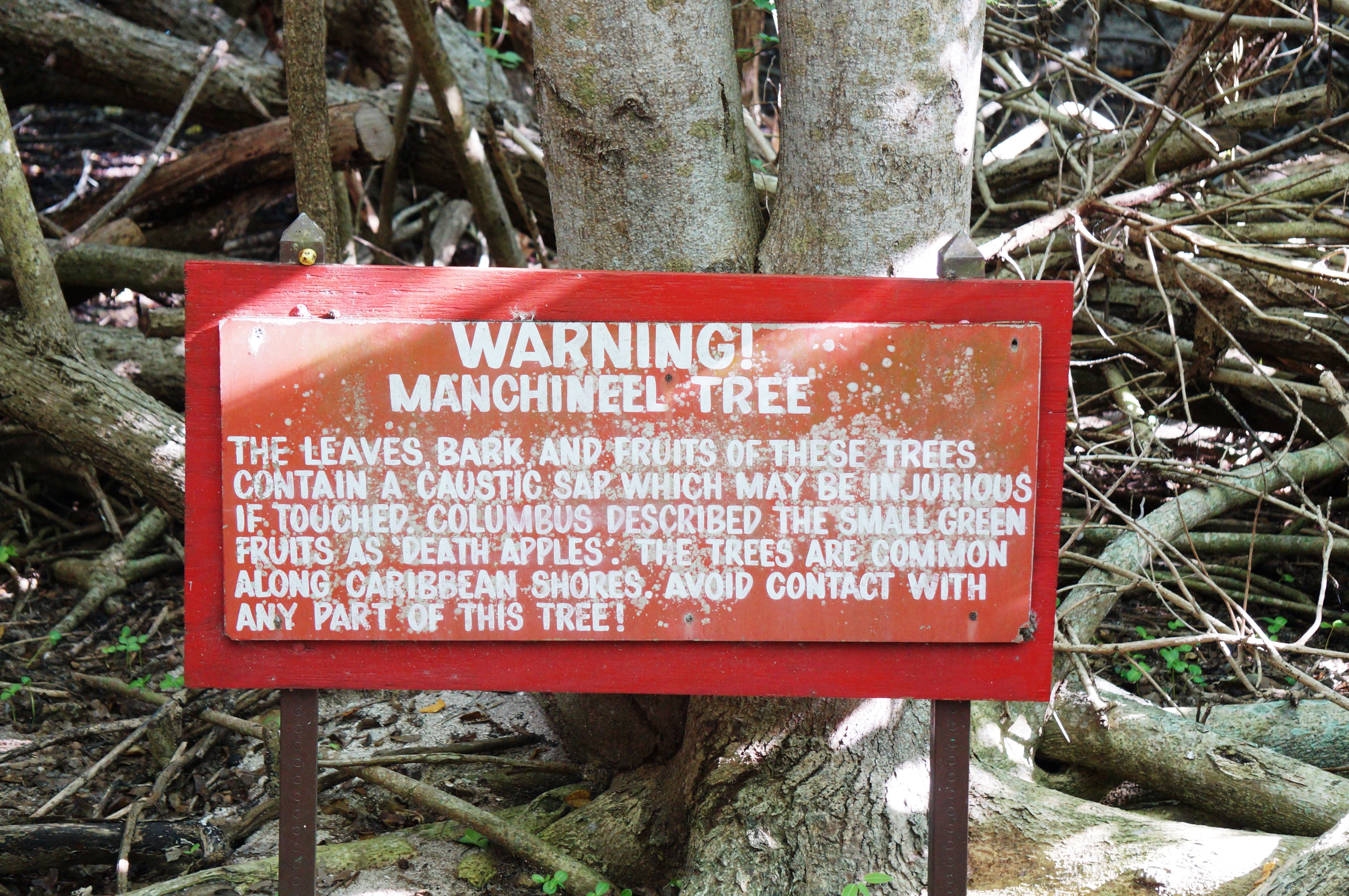This image captures an outdoor scene focused on a prominent red warning sign set against a backdrop of tree debris. The sign, which appears weathered and somewhat faded, is mounted on brown posts that look rusted and aged. It warns about the Manchineel tree (misspelled "Mon chenille" in one account), stating in white capital letters that the tree's leaves, bark, and fruits contain a caustic sap that can be harmful if touched. It also mentions that Columbus described the small green fruits as "death apples." Surrounding the sign is an area filled with various branches and tree stumps, with a truncated tree trunk visible, devoid of leaves and branches. The tree debris varies in thickness, suggesting that some branches have been recently cut off. This hazardous tree is common along the shores of the Caribbean, and the sign explicitly advises avoiding any contact with it. The overall scene has a rustic and somewhat neglected appearance, emphasizing the potentially dangerous nature of the environment.